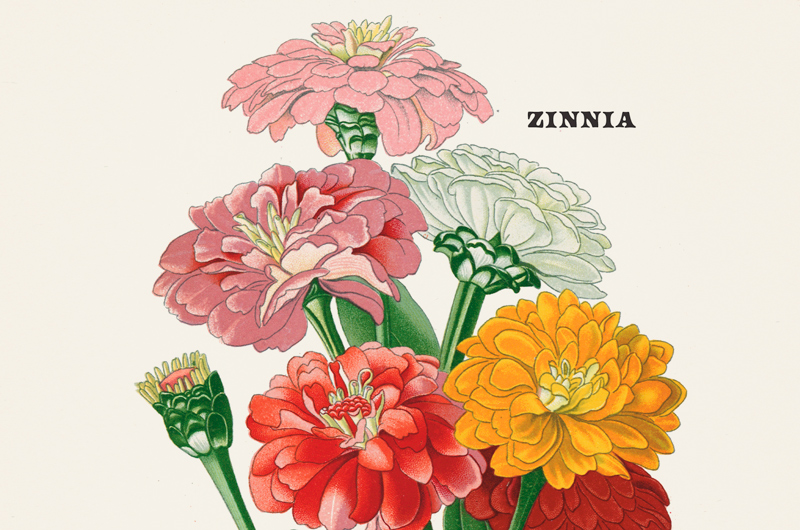The image presents a detailed, hand-illustrated graphic of Zinnia flowers against a white background. At the very top, a single pink Zinnia with yellow at its center stands tall. Below it, two more flowers flank it: pink on the left and right with yellow centers, and a white Zinnia facing away from view. Toward the bottom center is a vibrant red Zinnia, with another, darker red Zinnia slightly beneath it. To the bottom right, an orange Zinnia blooms, and to the bottom left, a flower in an early bud stage with green parts and an undeveloped center. All the flowers are drawn with green stems. The text "ZINNIA" appears in bold, all-caps serif font in the top right corner, closely integrated with the floral illustrations.